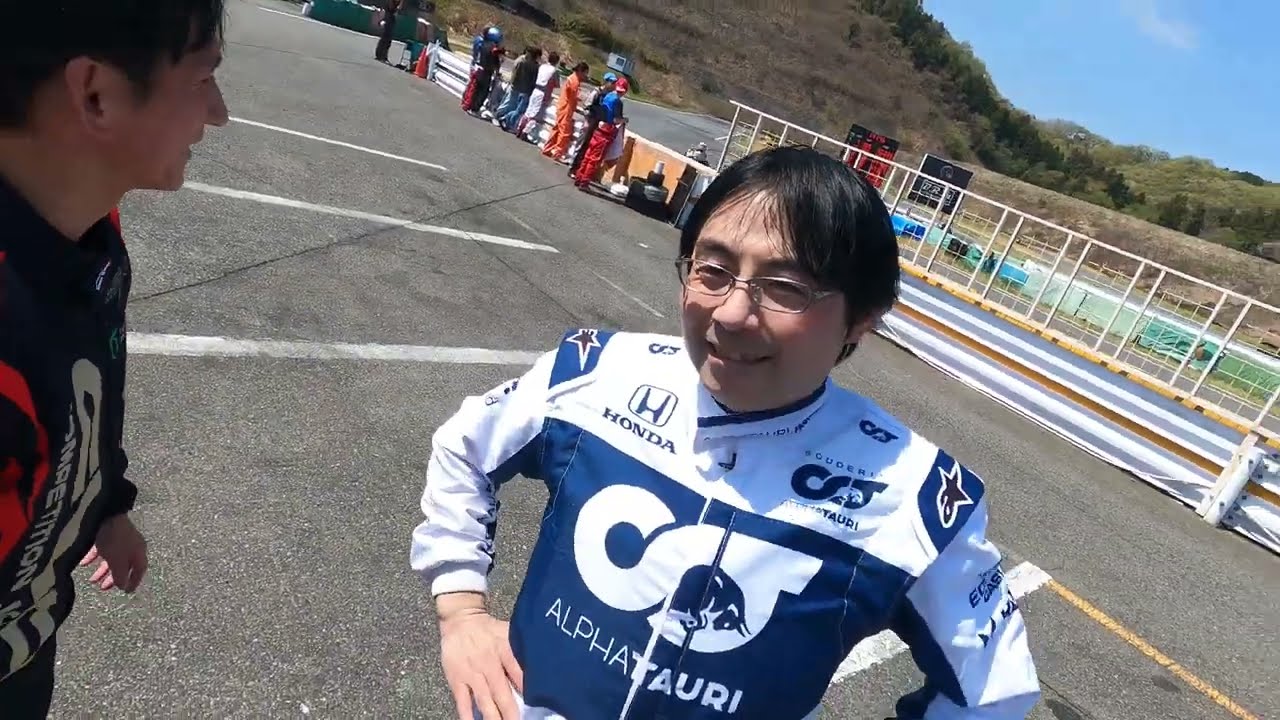This landscape-oriented photograph captures an Asian man, likely in his 30s or 40s, standing at the center of a racetrack scene. He has straight dark hair, glasses, and is joyfully smiling directly at the camera. He is wearing a white and blue long-sleeve racing shirt adorned with various logos, including Honda and AlphaTauri, along with stars on each shoulder. To his left, partially cut off, is another man with a profile view; he is also smiling and is clad in a white, black, and orangish-red racing shirt. 

The backdrop reveals a bustling racetrack environment. Concrete flooring with white and yellow lines marks the track, which is bordered by guardrails behind which several spectators stand, their backs turned as they face the track. Distant foliage, landscaping, and hills—some brown with green trees—stretch out beneath a blue sky dotted with light clouds in the upper right corner, illuminating the scene with bright daylight.